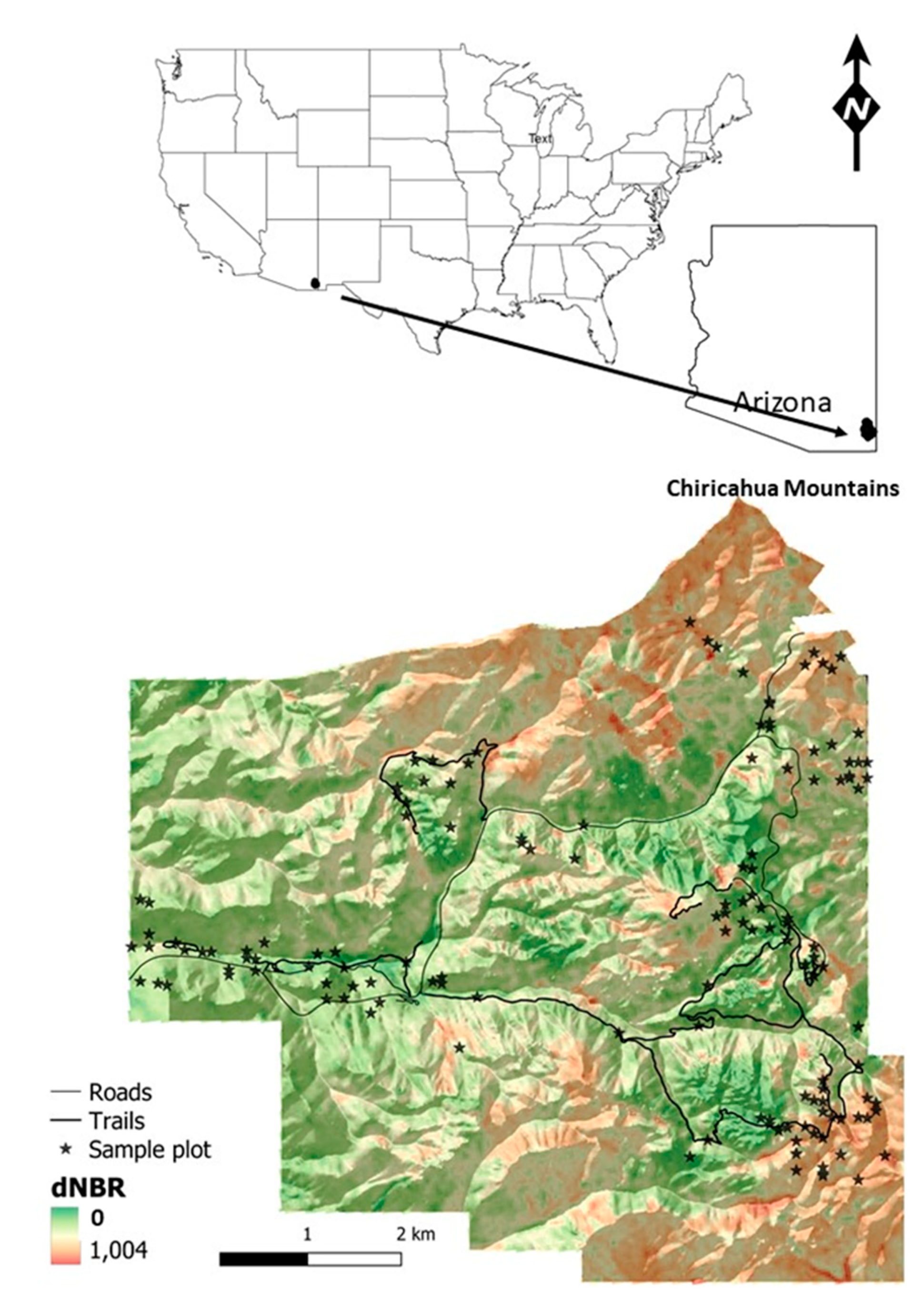The image starts with a simple, black and white map of the United States at the top, with clearly defined state borders but no text or labels. An arrow leads from Arizona in the bottom right corner of the map to a larger, detailed black and white outline of the state, highlighting the Chiricahua Mountains with a small cluster of black dots and labeled text. Below this, there is a detailed topographical map of the Chiricahua Mountains area, color-coded with gradients of greens, golds, and oranges. This map includes a legend in the bottom left corner that explains the color-coding and symbols: thin black lines for roads, thick black lines for trails, and black stars for sample plots. Additionally, there's a distance scale, further detailing the mountainous terrain.